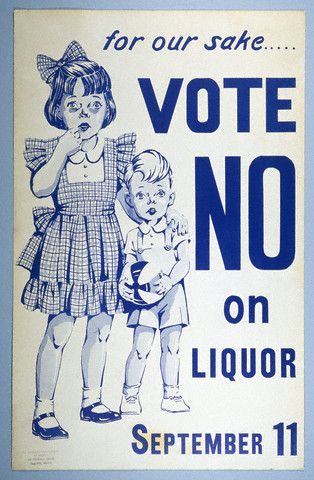The image is a tall, vertical sign with a light blue border and a white center that slightly ages into a beige color at the corners. It features a blue line illustration of two children— a young girl and a younger boy— standing together. The girl, who has a bob hairstyle and a ribbon in her hair, is dressed in a plaid jumper with puffy shoulders over a white collared blouse. She is wearing black shoes and white socks. The boy, positioned to the right of the girl, is in overall shorts and a white shirt, white shoes, and is holding a ball. Both children have wide eyes and concerned expressions, giving an impression of innocence and worry. At the top of the sign, in blue text, it reads, "For our sake..." followed by "VOTE NO" in larger, bold letters, and then "on liquor, September 11th" below it. The illustration and text together convey the message strongly, aiming to influence a vote against liquor.